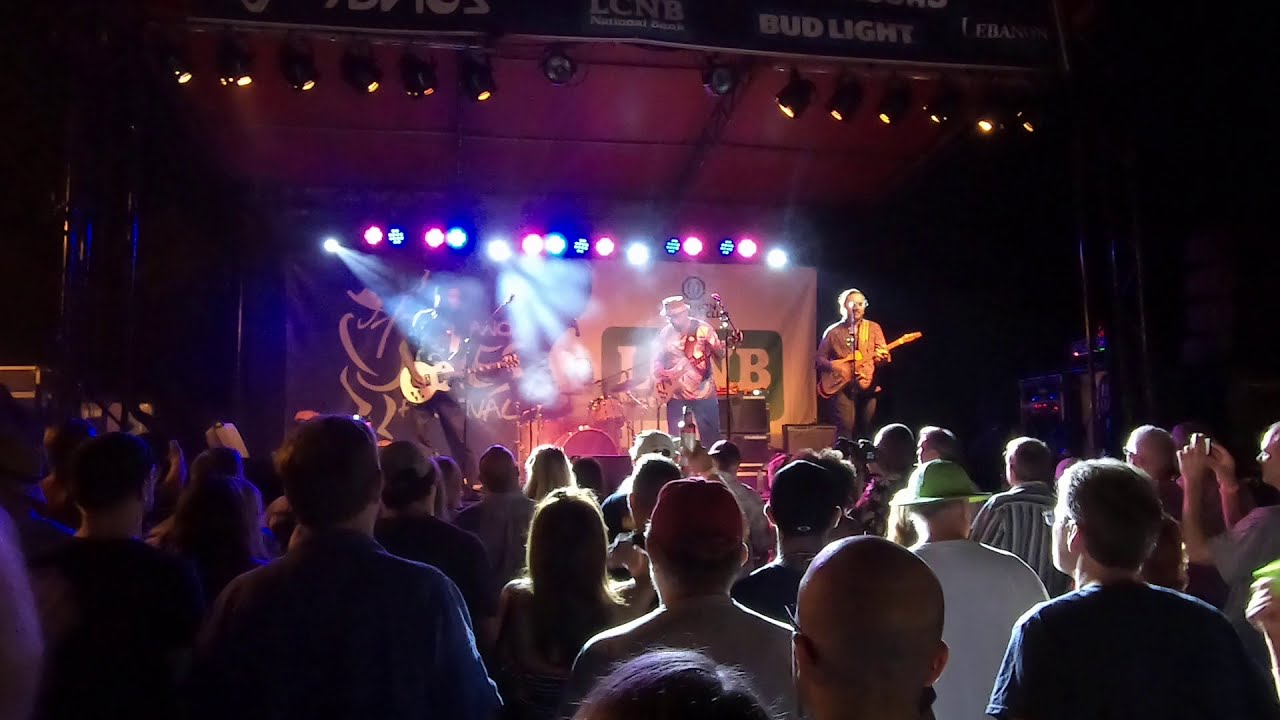The image captures a live concert featuring three men at the front of the stage, all playing guitars. The center of the stage is brightly illuminated by reddish, blue, and white lights that create a striking visual impact against the fog from a fog machine. Overhead, spotlights aim at the performers, enhancing their visibility. The middle musician, wearing a tan bowler's hat, tan shirt, and blue jeans, plays a tan guitar. To his left, a black man in a black shirt plays a white guitar, and to his right, a white man in a brown jacket and black pants plays a brown guitar. Each musician is equipped with a microphone.

Behind them is a set of drums without a drummer currently playing. The background stage area is dark, with several advertising signs visible above, including a Bud Light sign and partially obscured banners that might be sponsors. One banner possibly reads "National Bank."

In the audience, about two dozen people enjoy the performance, some capturing the moment with their phones. One person raises a beer bottle, perhaps in admiration or respect. The crowd, dressed in various outfits including one individual with what appears to be a green or yellow safety hat, shows an enthusiastic and engaged response to the music.